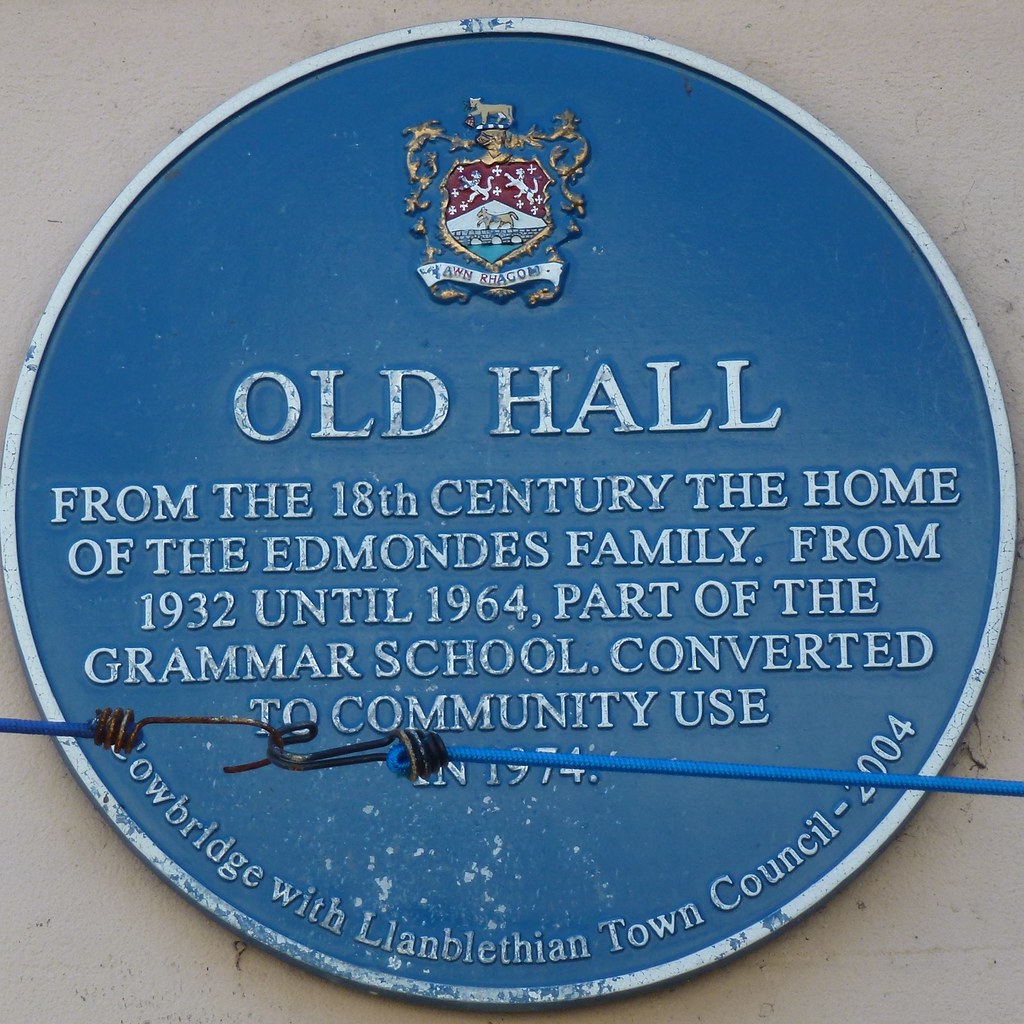The photograph captures a close-up of a historical marker outdoors, affixed to a gray stone wall. This large, circular blue metal plaque with a light gray rim spans most of the image. Prominently displayed at the top center of the plaque is a detailed family shield: the top half is red featuring two horizontal lines, while the bottom half is white, depicting a stone bridge over water with a goat walking on it. Above the shield, there's another smaller goat, and beneath it lies a decorative gold filigree design. Further down, the shield is complemented by a white banner inscribed with "AWNRHAGOM." The plaque's main body contains historical information in raised white lettering. It reads, "Old Hall from the 18th century, the home of the Edmonds family from 1932 until 1964, part of the grammar school converted to community use in 1974." At the bottom of the plaque, it states, "Cowbridge with Llanblethian Town Council, 2004." A pair of blue bungee cords with metal hooks is stretched horizontally across the bottom fourth of the plaque, likely serving to secure or demarcate it.